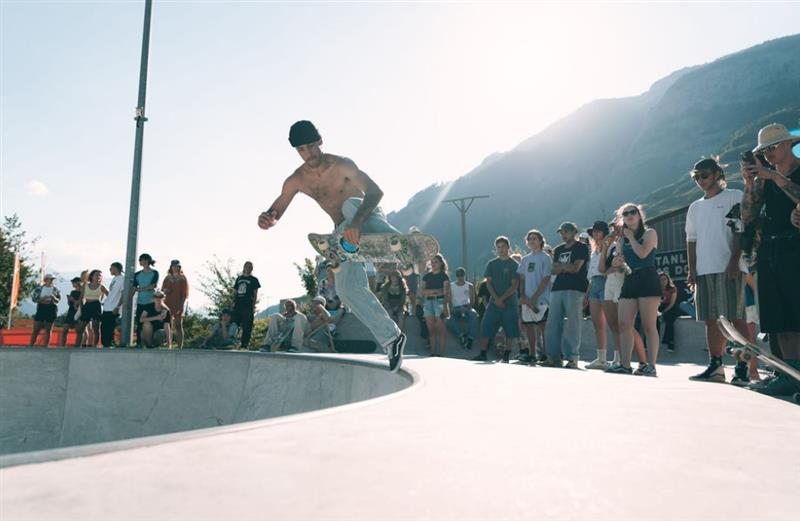The image captures an outdoor scene on a bright day in a skate park situated in a country-like desert mountainside. People dressed in summer attire—hats, shorts, and tank tops—are gathered around a large, concrete skate bowl, reminiscent of an old swimming pool repurposed for skating. The focal point is a shirtless Caucasian skateboarder with a black beanie and light blue jeans, performing a trick. He is mid-air with his left hand gripping the skateboard, which is adorned with various graffiti, inkings, stickers, and a notable blue circle. His right hand is extended outwards for balance while his right leg dangles and his left foot maintains minimal contact with the edge of the bowl. The backdrop includes a clear, light sky and steep mountains, with the sun glowing brightly above, highlighting the building just below the peaks. The scene is filled with onlookers enthusiastically capturing the moment on their phones.